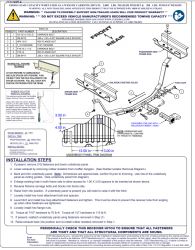This is a small rectangular image of an instruction manual, taller than it is wide, set against a white background and bordered by a thin gray line. The top features a wide gray rectangle containing a yellow triangle with a black exclamation point, indicating a safety warning. To the right of this warning are several rows of black and gray text, although they are not legible due to the small size and blurriness of the image. Below the text is a table consisting of four columns. To the right of the table, black diagonal text can be seen, though the content is unclear. Underneath, on the right side, are intricate diagrams of silvery metal objects, resembling metal brackets or components being assembled with screws. To the left of these diagrams are three smaller rectangular white shapes containing black or blue text. The overall layout and content suggest that the page provides installation steps for assembling a product, likely involving metal parts, although the exact details remain indistinct.